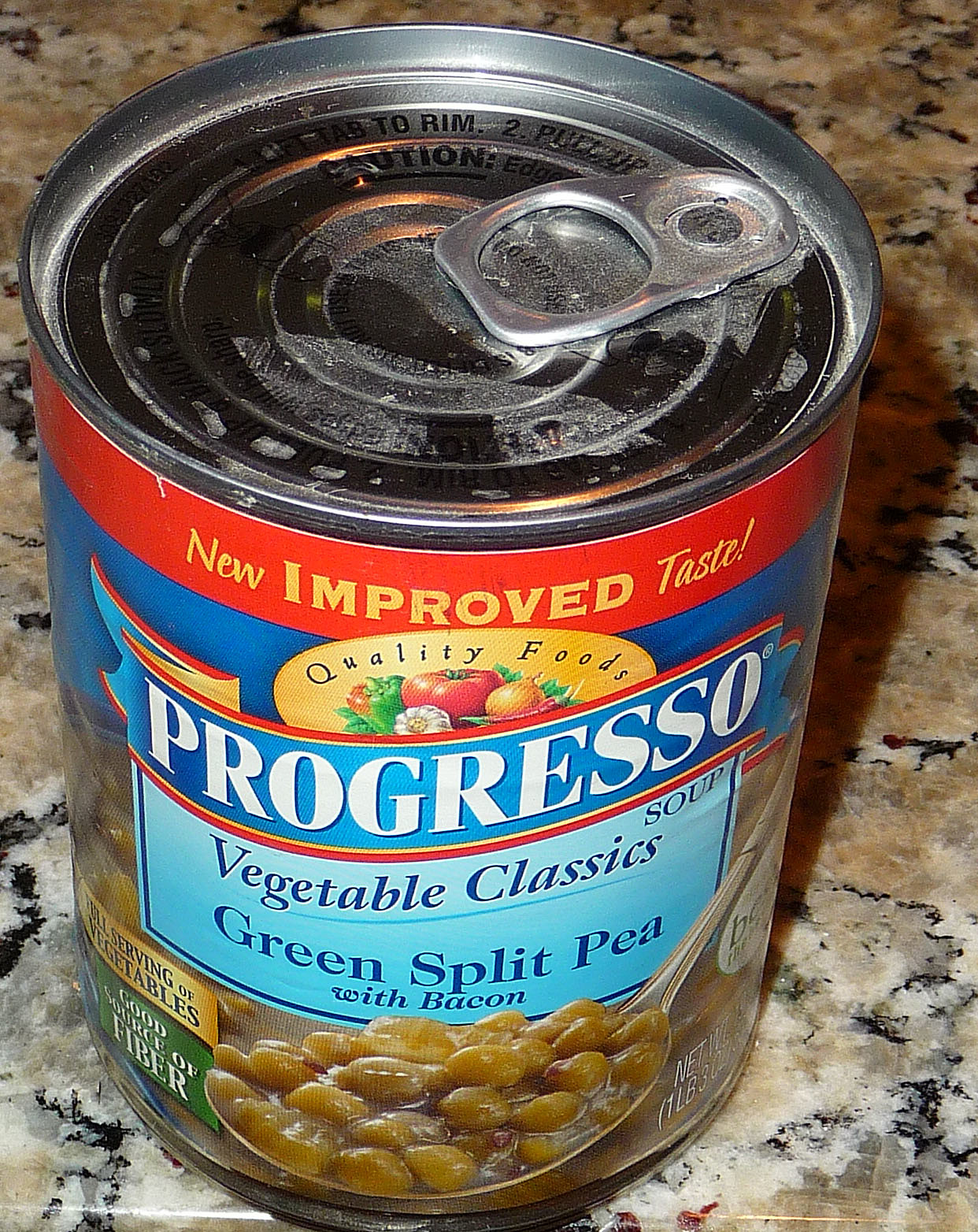The image features a can of Progresso Vegetable Classics Green Split Pea with Bacon soup. The photograph is taken from a slightly top-down angle, showcasing both the top lid and the full front label of the can. Positioned against a marbled granite surface, the background features a mix of light brown fading into dark brown tones, accented with hints of red and black striations. 

The can's label details include a prominent "New Improved Taste" banner in yellow with a red line border across the top. Beneath this, a header with the Progresso logo is displayed, where the brand name "Progresso" is emblazoned in white over a blue flag-like banner, accompanied by illustrative images of garlic, tomatoes, and onions, emphasizing the quality of ingredients. 

The main label reads "Vegetable Classics Soup" and highlights the "Green Split Pea with Bacon" variety. The visual depiction of the ingredients on the label shows split peas in their characteristic green hue, alongside small bacon pieces. Notably, the top of the can appears to have accumulated some residue, suggesting it has been stored in a pantry for an extended period.